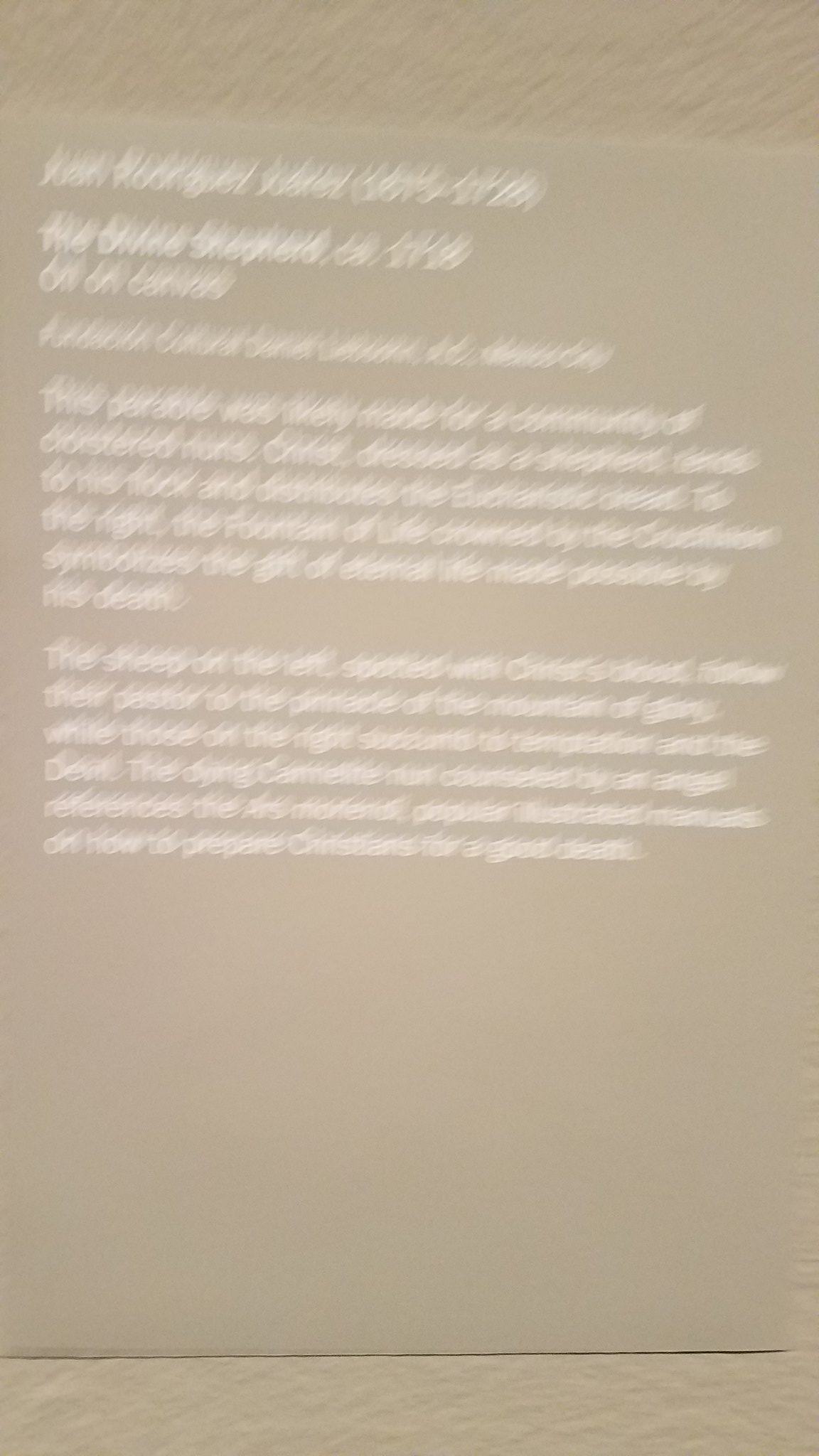The image depicts a very blurry plaque displayed against a white wall, with white text that appears almost 3D and difficult to read, creating an illusion reminiscent of looking through a drunken haze. The plaque, attributed to Juan Rodriguez Juarez, features the title "Divine Shepherd" at the top. Below, two paragraphs in small, white text detail a religious narrative: the left side recounts sheep spotted with Christ's blood and guided by a pastor to the pinnacle of glory, while the right side describes sheep succumbing to temptation and the devil, with a reference to preparing Christians for a good death. The plaque seems to be mounted on a gray, cushion-like background, adding to the overall subdued aesthetic.